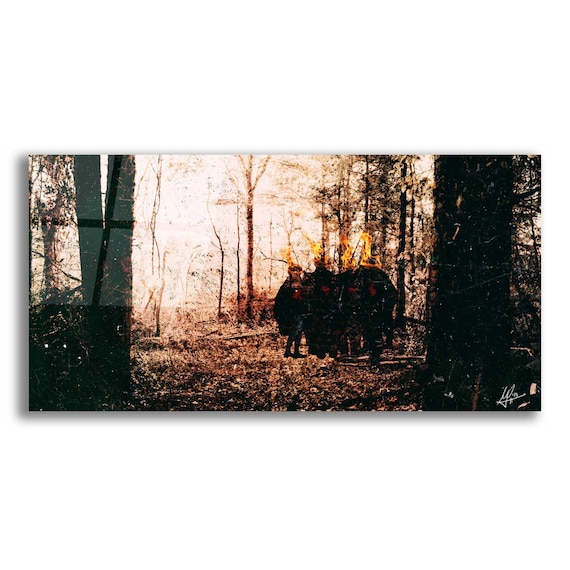This image captures a dark, atmospheric scene in a forest, characterized by several trees with sparse or no leaves. Dominating the right side, there's a large, thick tree trunk, while the left side features another sizeable tree trunk that splits into two further up. In the background and throughout the middle of the image, smaller, thinner trees are scattered. The entire scene has a muted color palette ranging from browns to blacks, suggesting an old, somewhat rumpled photograph.

In the middle ground, slightly off-center towards the right, there appear to be four indistinct human figures standing together. Due to the poor quality of the photograph, their faces are not visible; instead, their heads are oddly depicted with flames or fire-like visuals. Their feet, facing towards the viewer, are vaguely discernible. 

Additionally, there is a faint overlay of what looks like a window grid on the top left side of the image, adding an eerie, surreal element to the composition. On the right edge of the photo, there's a barely legible white signature, adding to the mysterious nature of the scene. The overall impression is that of an old, haunting photograph of four people in a forest, with their heads seemingly on fire, enveloped by a shadowy, melancholic ambiance.